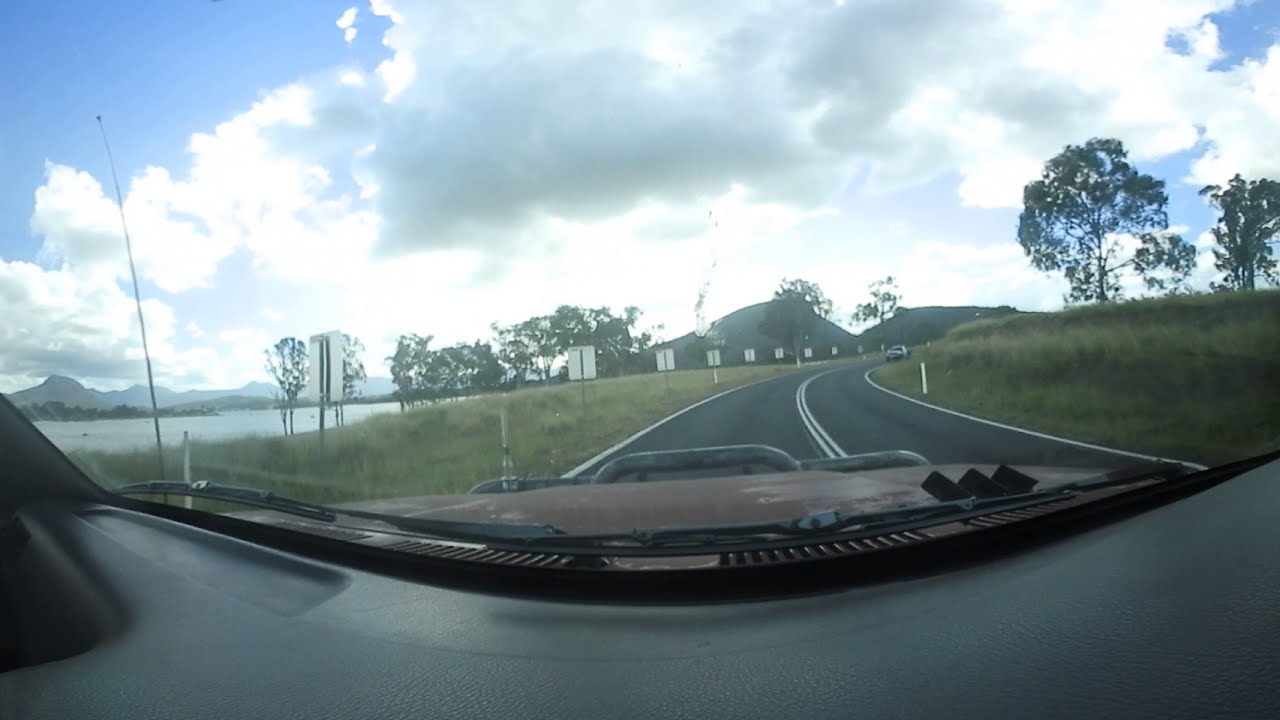The image is a distorted fish-eye view taken from inside a vehicle, capturing the scene through the windshield. The foreground displays the vehicle's black dashboard with visible windshield wipers and a small part of the grill and bumper. There’s even an antenna on the left side of the hood. The road depicted is a two-lane highway with solid yellow lines, curving slightly to the right as it extends into the distance. Alongside the road, there are grassy fields on both sides with a mix of green and brown grass.

On the left, the grassy field borders a large body of water with a strip of shoreline, and in the far distance, a line of dark mountain peaks. On the right side of the image, more grassy fields and a few trees are visible close to the horizon. There is another car on the road, driving toward the viewer from the point where the road starts to curve. The overall sky is a mix of light and dark blue, heavily overcast with various cloud formations that cover about three-quarters of the sky, giving the scene a somewhat gloomy atmosphere.